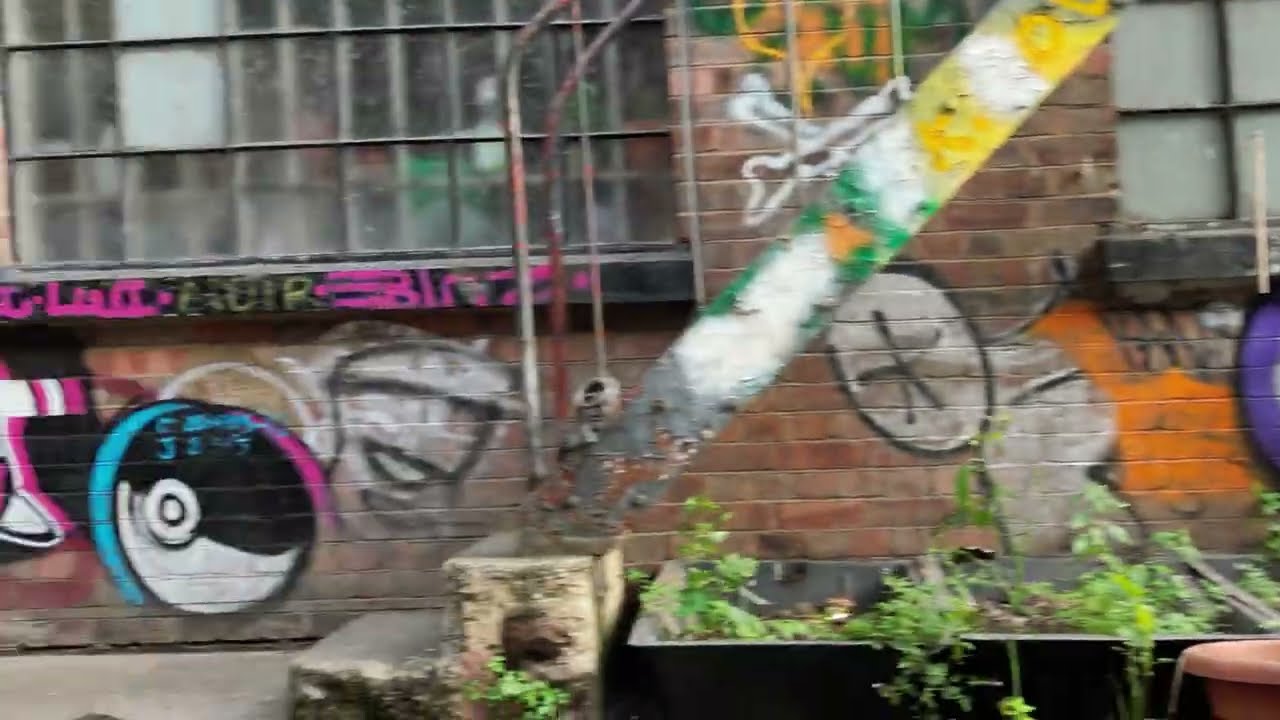This photograph captures a close-up of the side of a brick building adorned with vibrant, colorful graffiti. Dominating the scene is the outer wall of the building, which features an array of spray-painted artwork. On the left-hand side, a graffiti image resembling a black and white Pokéball, highlighted with bright turquoise blue and pink accents, stands out. Below this, various other graffitis, including shapes in colors like black, white, pink, blue, green, yellow, and orange, cover the bricks.

The building also has two prominent windows: a larger one on the top left and a smaller one on the top right, both of which appear dirty and obscure any view inside. The exterior wall's graffiti continues around these windows. Below the wall, two gray concrete steps lead upwards to the right, connecting to a metal staircase painted with splashes of white, green, orange, and yellow. These stairs exhibit signs of weathering and additional graffiti.

At the bottom right, a black rectangular planter houses some green plants, accompanied by a small, partially visible red terracotta pot further right. The overall scene appears to be a street or walkway adjacent to the exterior of a building, characterized by its urban and slightly neglected atmosphere.